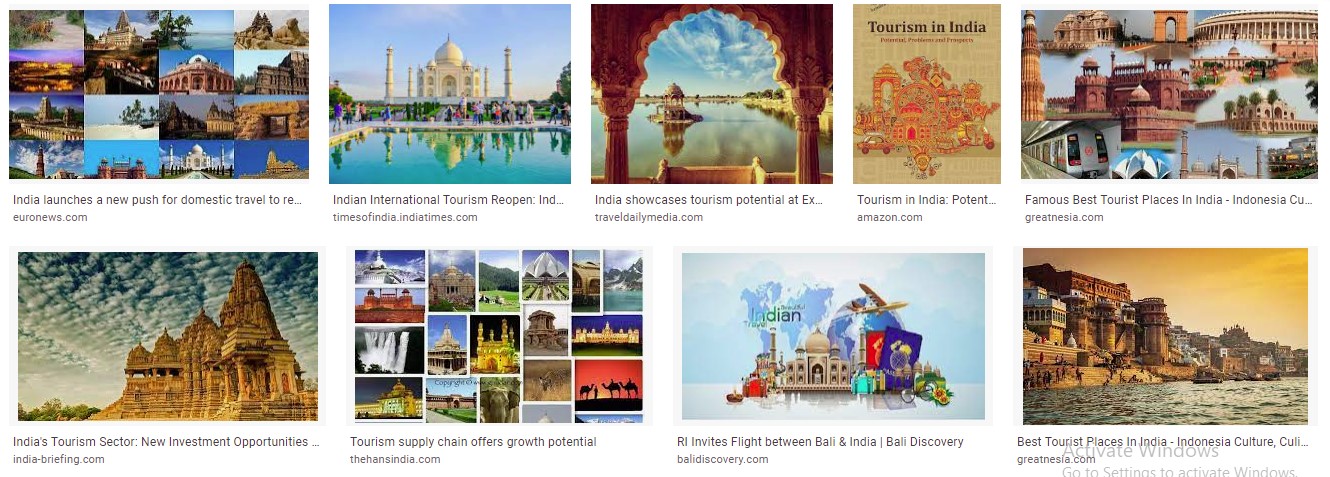A screenshot capture showcases the search results for "tourism in India," presumably from Google Images or a similar browser-based image search. The screen comprises 9 distinct photographs encapsulating various aspects of India's rich and multifaceted tourism sector.

- **Top Left:** A collage of architectural marvels from India captioned, "India launches a new push for domestic travel."
- **Top Center:** An elegant illustration of the iconic Taj Mahal, with the caption, "Indian international tourism reopens."
- **Top Right:** A photo taken from within an outdoor corridor of a historical building, captioned, "India showcases tourism potential."
- **Middle Left:** This image resembles a detailed book or guide, featuring an intricate illustration and captioned, "tourism in India."
- **Middle Center:** A creatively edited montage of famous tourist destinations in India, captioned, "famous best tourist places in India."
- **Middle Right:** An image related to India's tourism industry developments, titled "India's tourism sector, new investment opportunities."
- **Bottom Left:** Represents opportunities in the tourism supply chain, captioned, "tourism supply chain offers growth potential."
- **Bottom Center:** Highlights international travel connections with a title, "R.I. invites flight between Bali and India, Bali discovery."
- **Bottom Right:** Depicts cultural aspects with the caption, "best tourist places in India, Indonesia culture."

Each image is thoughtfully captioned to reflect various enticing facets of Indian tourism, from majestic landmarks and cultural insights to business opportunities and international travel initiatives.